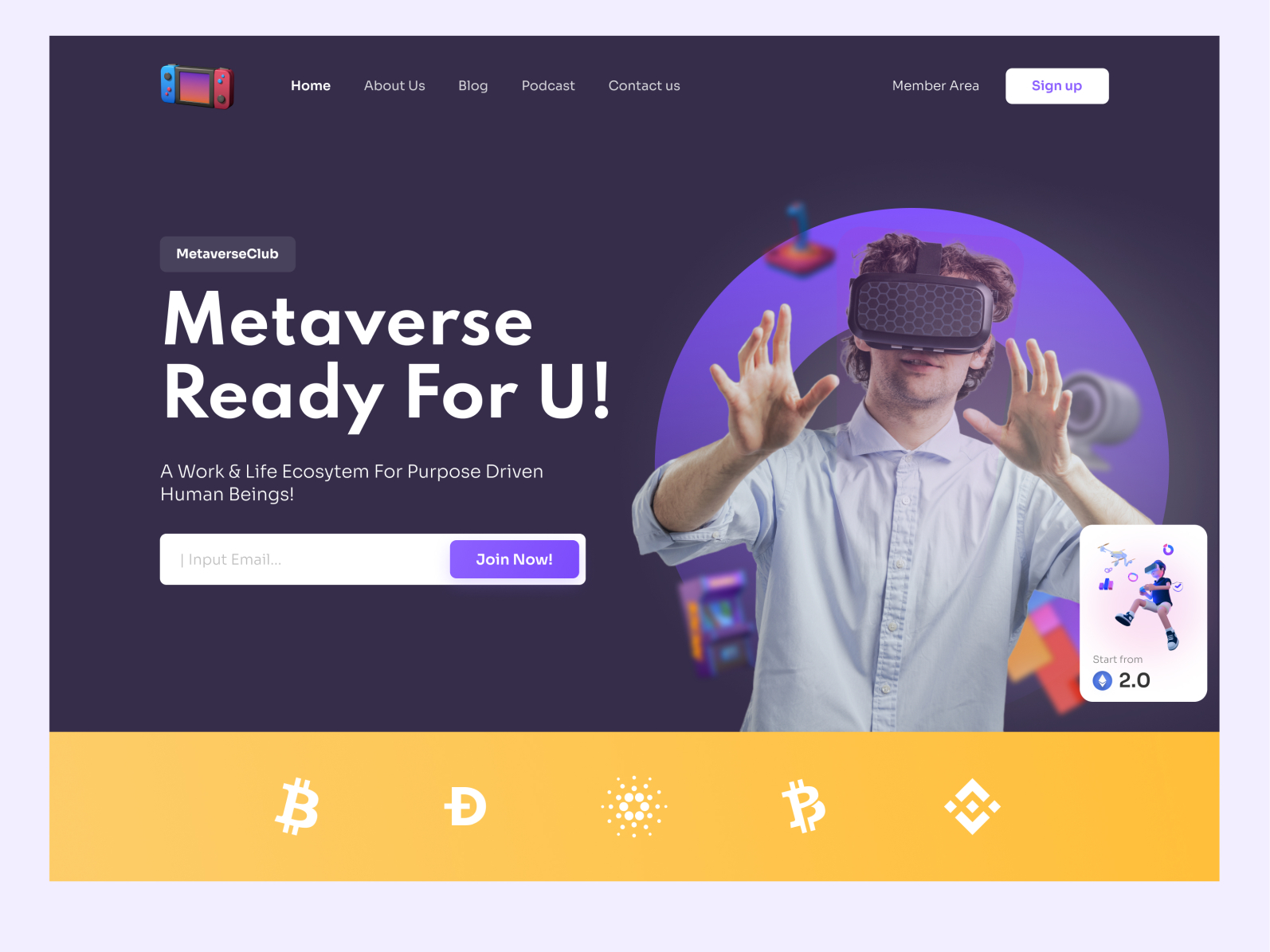This is a detailed caption for the described image:

The screenshot appears to be of a website or an advertisement, featuring a light purple border surrounding the main content. The central section of the image is dominated by a dark purple box at the top and a bright yellow banner at the bottom. 

In the top left corner of the dark purple section, there is vector art of a Nintendo Switch, next to which is the bolded white text "Home," indicating the current page. Following this, the menu options "About Us," "Blog," "Podcast," and "Contact Us" are also in white but not bolded. On the right side of the dark purple section, "Member Area" is written in white, and near it, there is a white button with purple text that reads "Sign Up."

Below this header is a dark gray rectangle with the title "Metaverse Club" in white text. Prominently displayed within the same rectangle, in large white letters, is the slogan "Metaverse Ready For You!" Beneath that, in smaller white text, it says, "A work and life ecosystem for purpose-driven human beings!"

Within this dark gray section is a white input box labeled "input email..." accompanied by a purple button to the right that reads "Join Now." Adjacent to these elements, there's a high-resolution image of a person wearing VR glasses, with a stylized circular design and vector art elements in the background. Additionally, in the bottom right corner of this section, there is an avatar illustration also wearing VR glasses, with the text "Start from 2.0" beneath it.

The yellow banner at the bottom includes several cryptocurrency symbols: a Bitcoin symbol, a "D" symbol, another cryptocurrency icon with dots extending out from its center, a second Bitcoin-like symbol, and a diamond-shaped symbol.